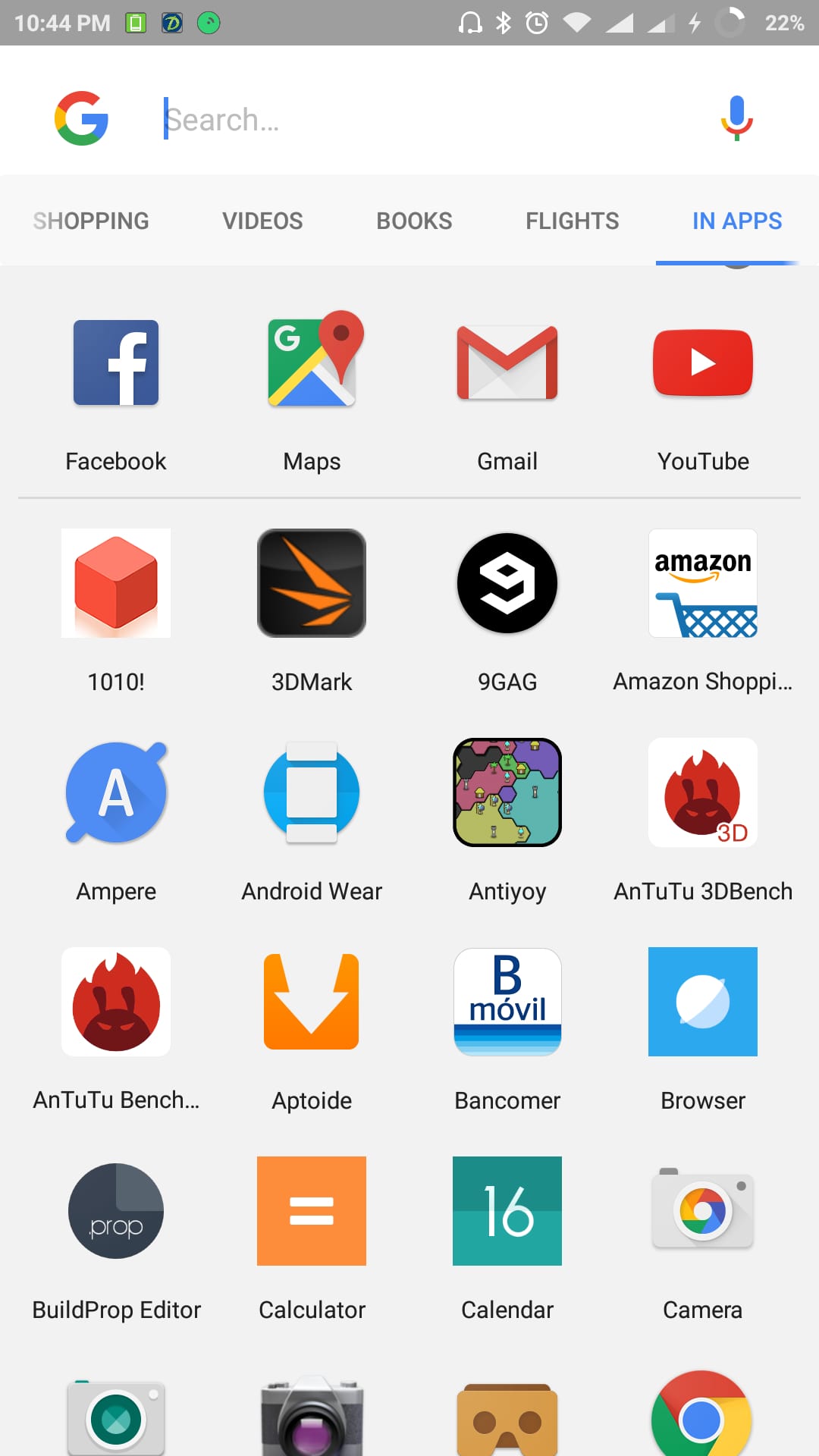This detailed caption describes a screenshot of an Android phone's app drawer:

In this screenshot of an Android phone's app drawer, the display time in the upper left corner reads 10:44 p.m. The notification bar is populated with several icons, while the battery level in the upper right shows 22 percent. Below the notification bar, the area has a white background, featuring the colorful Google "G" logo on the far left. Adjacent to the Google logo is a search bar with light gray text that says "Search," and a microphone icon for voice search is positioned to its right.

The main section of the app drawer showcases all the installed applications. At the top of this section, the quick launch area includes icons for Facebook, Maps, Gmail, and YouTube. Beneath these quick access apps, an extensive list of applications is visible. Among them are apps such as 1010! with an exclamation point, 3DMark, 9GAG, Amazon Shopping, Ampere, Android Wear, AnTuTu, AnTuTu Benchmark, Aptoide, BBVA (Bancomer), Browser, BuildProp Editor, Calculator, Calendar, and Camera. Each app icon represents a shortcut that users can tap to launch the corresponding application directly from the app drawer. Numerous other apps are present but are not fully visible in this screenshot.